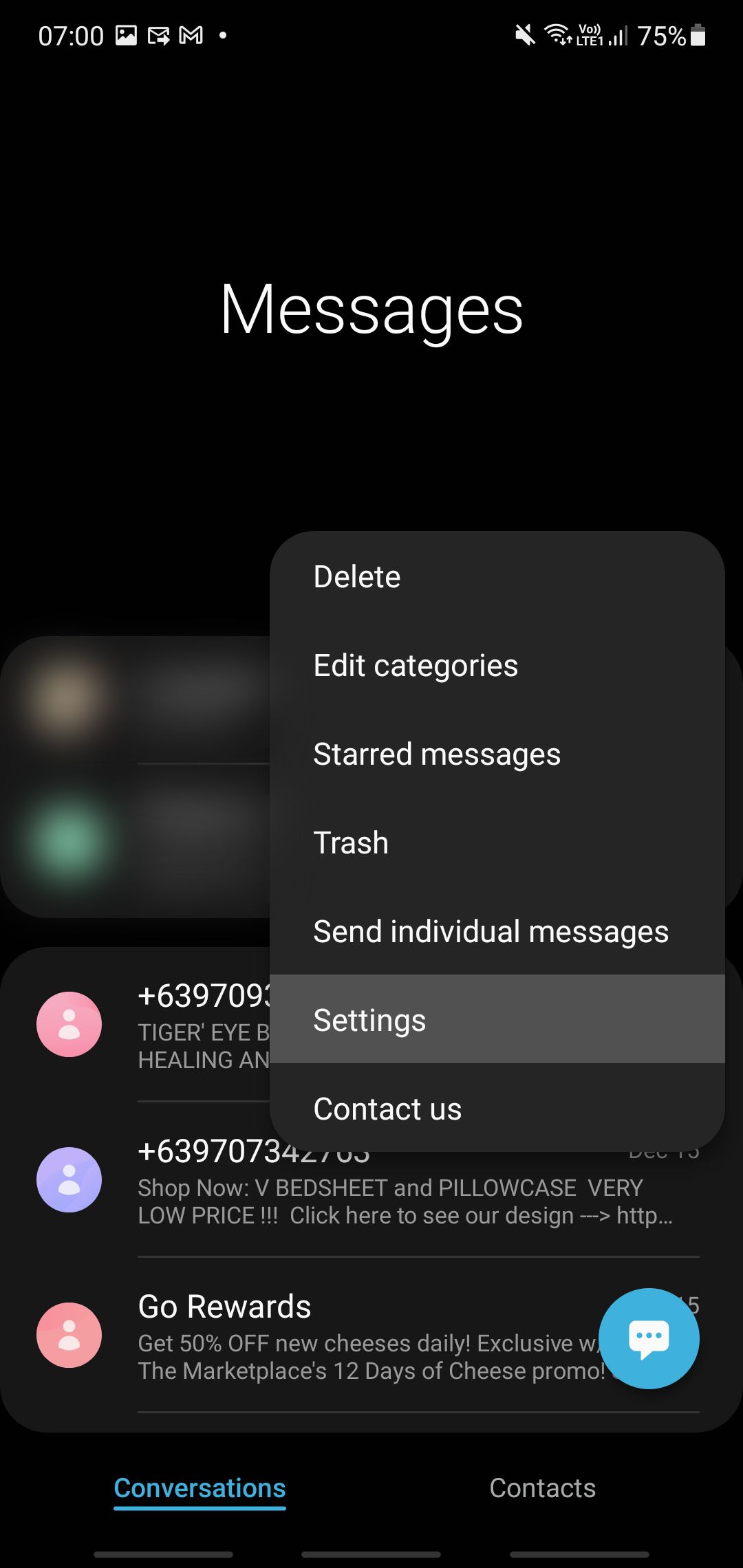The image features a black background at the top displaying the time as 7:00 o'clock, with indicator icons showing 3 or 4 signal bars and a 75% battery life. Below these indicators, in large bold white letters, the word "MESSAGES" is prominently featured. A grey pop-up menu appears underneath it, listing options such as DELETE, EDIT CATEGORIES, STAR MESSAGES, TRASH, SEND INDIVIDUAL MESSAGES, SETTINGS, and CONTACT US, with SETTINGS highlighted in a light grey box.

Partially visible in the background behind the pop-up menu is a series of elements. There's a string of digits, 639709, followed by the text "Tiger Eye Healing." Below this, a light blue oval encloses a generic profile picture with the number +639703 adjacent to it. The background also includes promotional text reading "SHOP NOW, THE BEDSHEET AND PILLOWCASE, VERY LOW PRICE, CLICK HERE TO SEE OUR DESIGN" and another message saying "GO REWARDS, GET 50% OFF NOW."